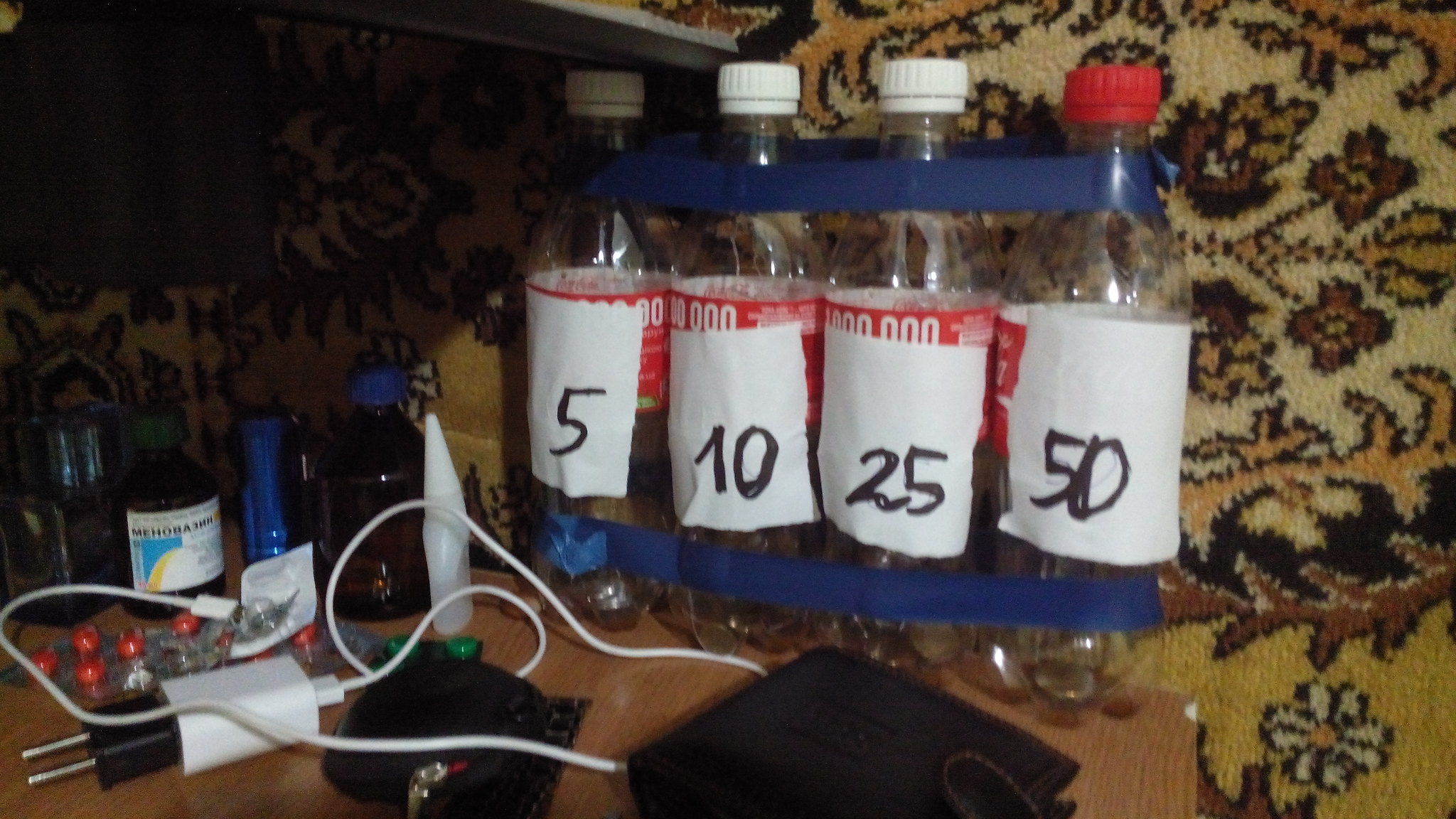This photograph captures a detailed scene centered around a light-colored wooden nightstand positioned on an ornate, beige, brown, and black Persian-style carpet featuring a floral pattern. The primary focus is on four plastic soda bottles, similar to Coca-Cola bottles, arranged side by side. These bottles are secured by blue painter's tape around the necks and bases. The first three bottles have white caps, while the fourth has a red cap. White pieces of paper, affixed to the bottles, bear black marker labels reading "5," "10," "25," and "50."

In front of the bottles, a black wallet is placed, with a white charging cable coiled to its left. The cable features a black plug with silver prongs. Further left lies a pill packet, partially empty, containing red pills. Adjacent to this arrangement is a section of the nightstand, which holds various other items, including bottles with different colored caps, hinting at a cluttered yet detailed snapshot of daily life.